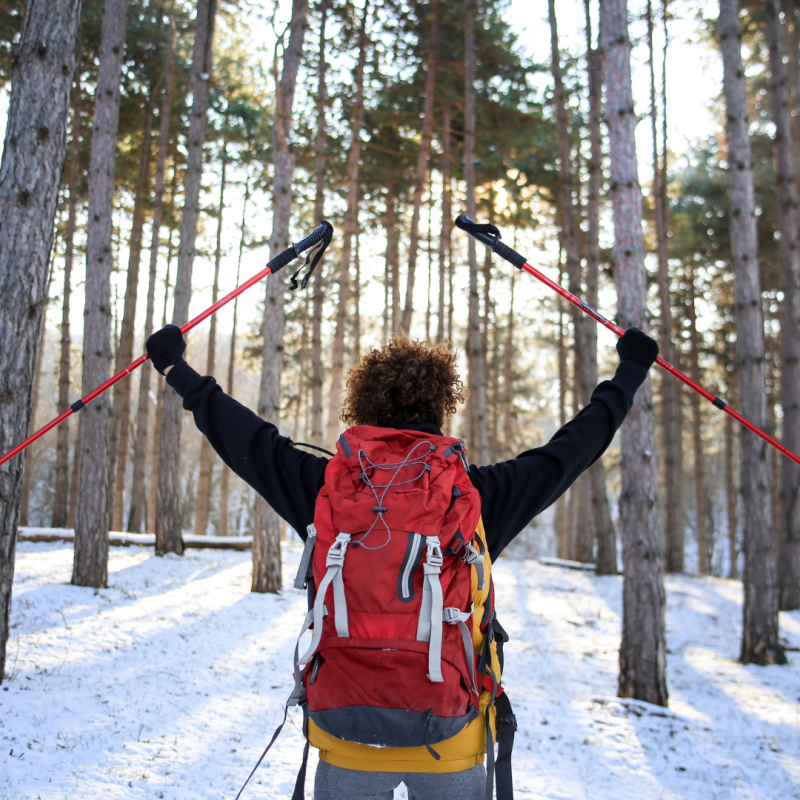In this winter outdoor scene, a skier is captured from the thighs up, standing in a snow-covered forest. The skier, viewed from behind, is wearing a vibrant red backpack with white straps, a black long-sleeve shirt with the bottom portion being yellow, and black gloves. His gray pants contrast with the winter setting. The skier has dark brown, curly, medium-length hair and is holding up his red ski poles with black handles in a triumphant pose, his arms outstretched above his head. The forest around him features tall, bare trees with light gray trunks, and in the background, the treetops hint at some greenery. The bright, clear sky adds a sense of crispness to the cold, snowy landscape.